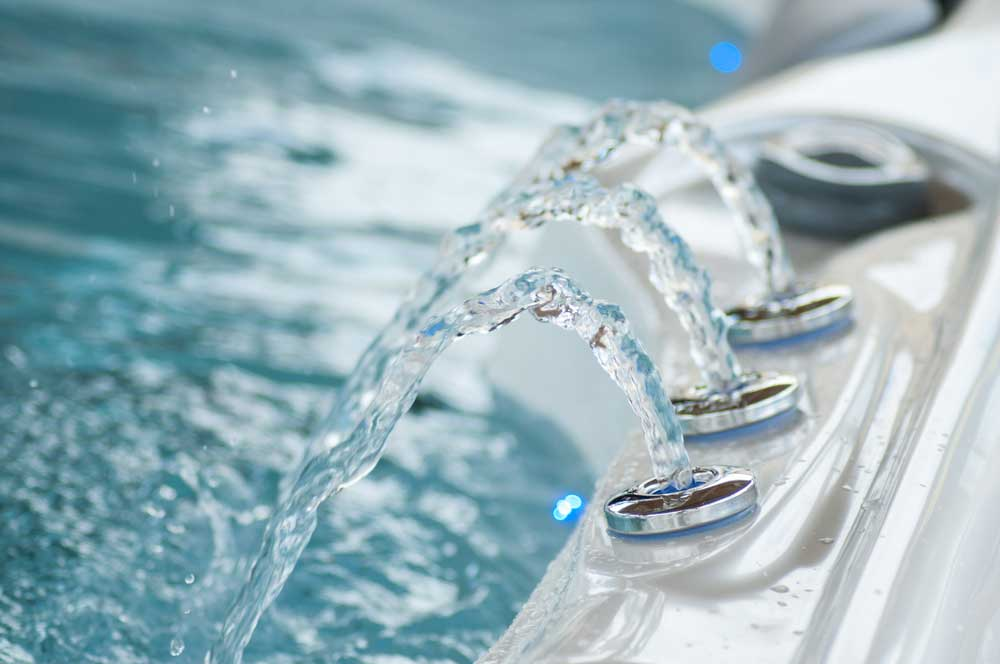The image displays the inside of a luxurious, modern jacuzzi tub. The tub itself is primarily white with a touch of gray and features a sleek, plastic finish. Three water spouts, appearing as round buttons, emit thick streams of water into the tub, creating a fountain-like effect. The water is exceptionally clear, with a greenish-blue tint, giving it a refreshing look. The spouts are positioned to provide a massaging effect, likely targeting a person's back, and are complemented by a noticeable larger button at the corner of the tub. The side of the jacuzzi, slightly blurred at the top, showcases the ergonomic curvature designed for comfort. Bright blue lights, likely indicating the jets or massaging features, add a touch of elegance and modernity to the tub's appearance.